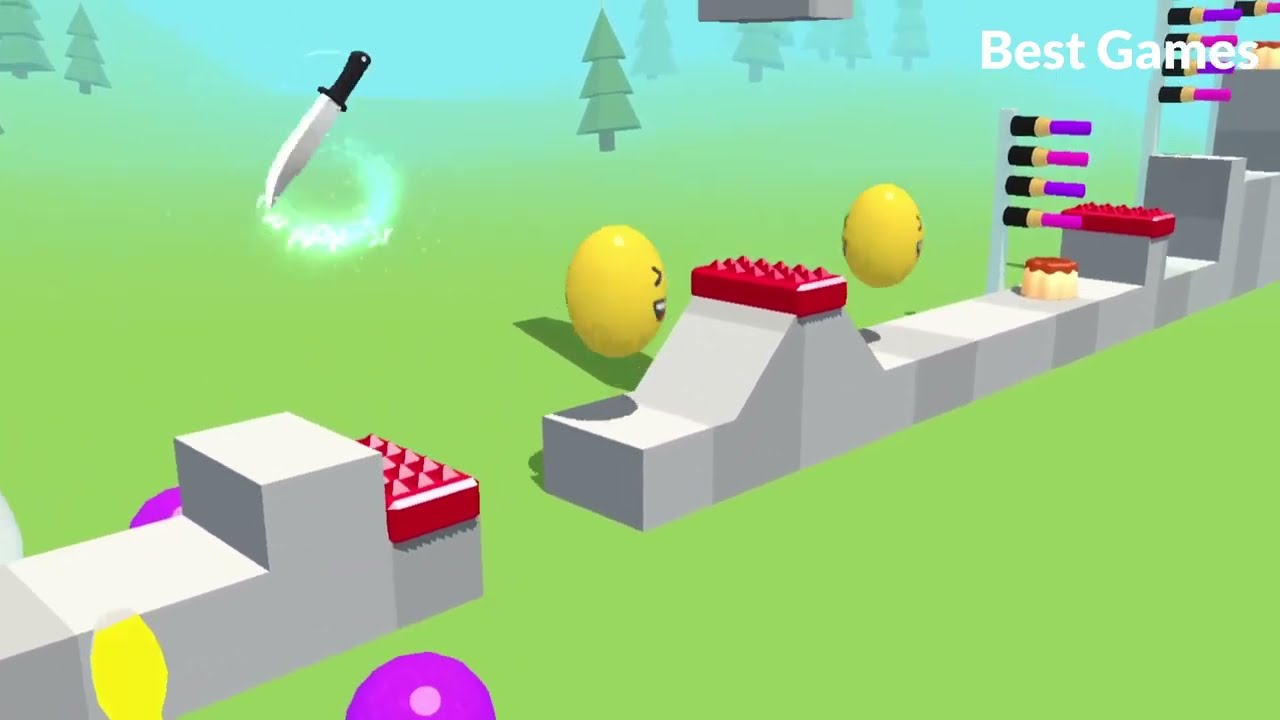The scene is a colorful, animated video game resembling a Lego block set intertwined with elements reminiscent of Pac-Man. The background transitions from green at the bottom to light blue at the top, adorned with multiple animated evergreen trees, creating a vibrant and dynamic setting. Dominating the scene are bouncing yellow balls with smiley faces, scattered behind an obstacle course that looks challenging yet inviting. The course features various red Lego blocks and gray walls in two shades of gray, alongside bars that likely need to be jumped over. Adding to the intrigue is a prominently placed knife with green and blue hues near the upper left, suggesting a potential weapon for the player. In the foreground, a shiny purple spherical object sits near the center-left, contrasting with the lively backdrop. The upper right corner displays the text "Best of Games" in white letters, reinforcing the gaming context. Overall, the main colors are green, blue, yellow, and red, creating a visually engaging and detailed environment.